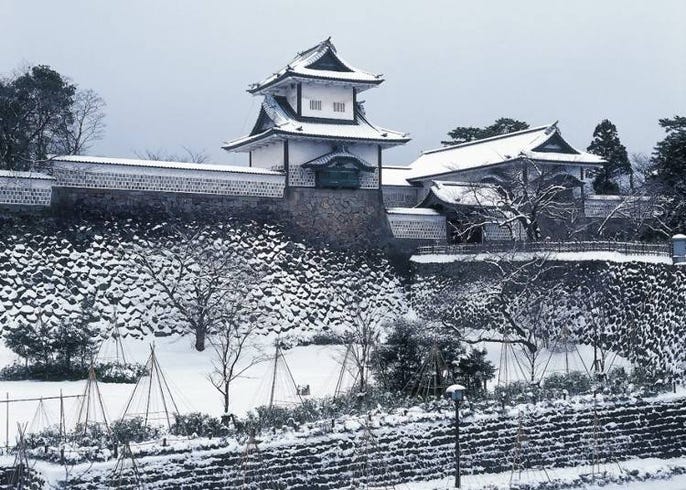This image showcases a traditional Japanese or Chinese temple perched majestically atop a steep, snowy hill. The temple features the iconic arched roofs with sharp peaks, characteristic of ancient East Asian architecture. The structure is built on a robust foundation of rock, with stonework forming a circular driveway around it. A high rock wall extends from beneath the temple, winding its way down the hill to a snow-blanketed field. A protective fence lines the wall, ensuring safety along the steep descent. Although the heavy snowfall obscures finer details, hints of a garden and a few trees peek through the white blanket, inviting the viewer to imagine the serene beauty that lies beneath. The background melds seamlessly with the temple, as the sky is a solid, snowy white, adding to the enchanting and peaceful ambiance of this winter scene.